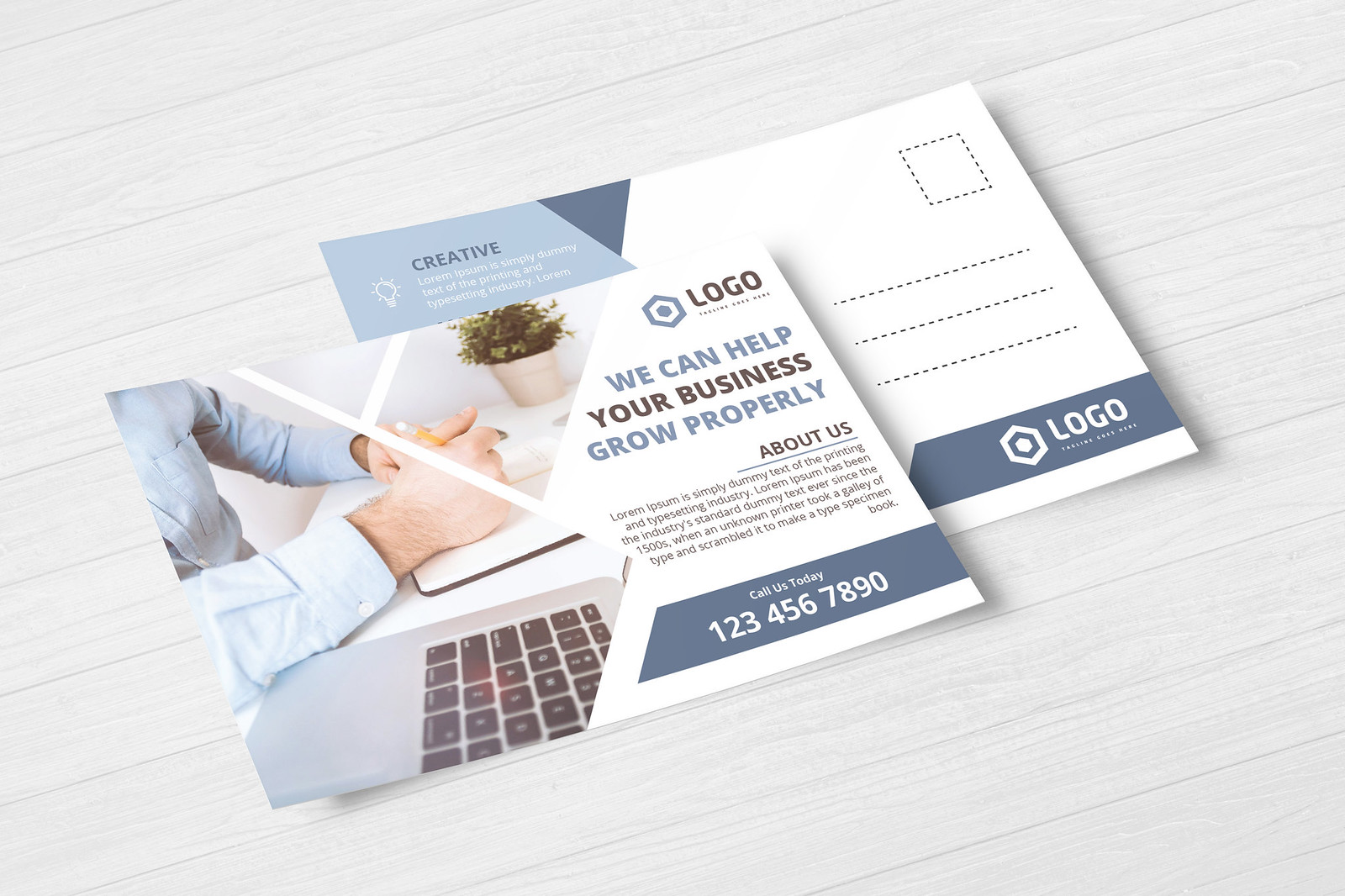The image shows an advertising brochure for a logo with the message, "We can help your business grow properly." It has two postcard-like items on a white table. The brochure also mentions a phone number, 1-234-567-890, and includes an "About Us" section, albeit in small, somewhat illegible text. One card depicts a person wearing a blue shirt, sitting at a desk, writing with a pen or pencil next to a tablet, a computer keyboard, and a potted plant. The second card, which looks like an envelope for mailing, features spaces for a stamp and an address, with "creative" written on the upper left. Both cards display shades of white and dark blue, surrounded by ample white space, suggesting a clean and minimalist design.